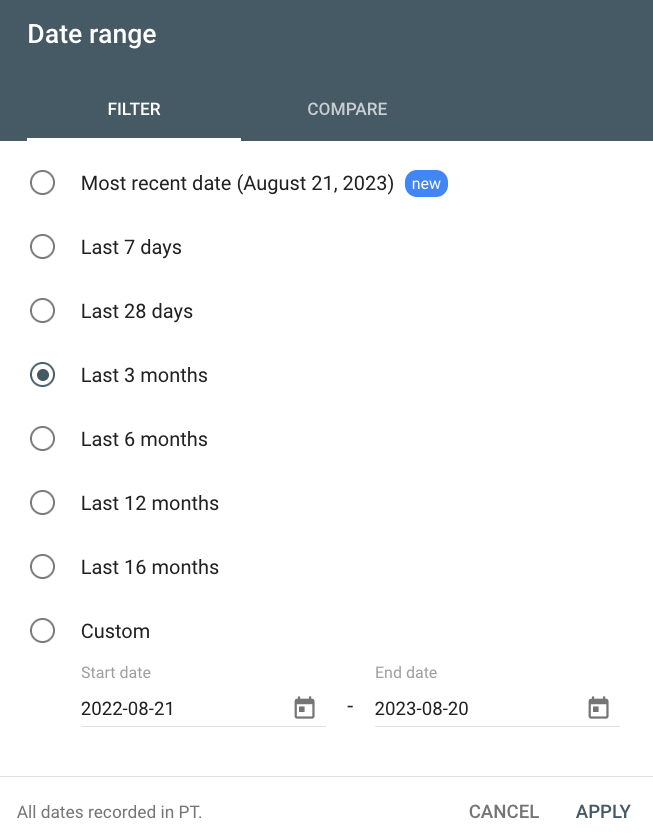The top section of the image features a prominent black rectangle. On the left side of this rectangle, the word "Filter" is displayed in white text, while the center of the rectangle features the word "Compare." Below this, on the left side, there is a vertical array of text with circles in front of each line. One of these circles contains a black dot, indicating selection. The first line reads "Most Recent Date: August 21st, 2023," and next to it, there's a blue oval-shaped button labeled "New."

Following this, there are several options with circles in front of them: "Last Seven Days," "Last 28 Days," which has a black dot within the circle indicating it is selected, "Last Three Months," "Last Six Months," "Last 12 Months," "Last 16 Months," and "Custom." Below this, the text reads "Order Date" with the date "2022-08-21" following it. To the right of "Order Date," the text "End Date: 2023-08-20" is displayed. At the bottom right corner of the image, there are two buttons: a "Cancel" button and an "Apply" button.